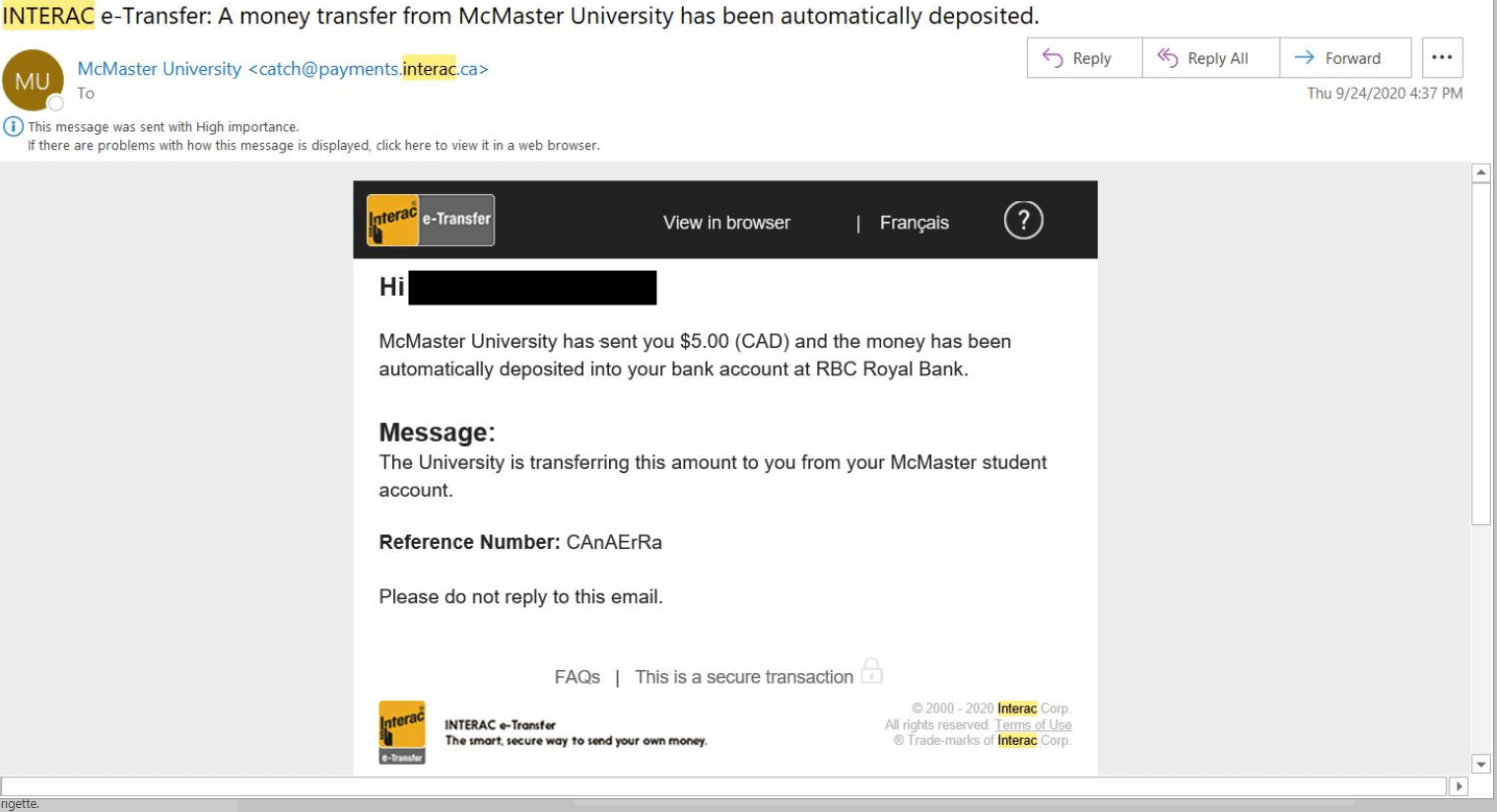The image is a screenshot of an email notification highlighting an e-transfer from McMaster University. At the very top, the word "Interact" is emphasized with a yellow highlight, and adjacent to it, "E-Transfer" is mentioned, indicating that a money transfer from McMaster University has been automatically deposited. The email interface includes buttons such as "Reply," "Reply All," "Forward," and an option represented by three little dots for additional actions. 

On the left side of the email, there is an avatar labeled "In the Unit" associated with the email address McMasterUniversityCatchAtPayments.Interact.ca. A timestamp is visible on the top right, showing the date Thursday, September 24, 2020, and the time 4:37 PM. 

The main message area features a black banner at the top, and a black box obscures a name, starting the message with "Hi." The body of the email reads that McMaster University has sent the recipient $50 CAD, which has been automatically deposited into their bank account at RBC World Bank. Additional content includes a reference number, an FAQ section, and the logos for Interact and E-Transfer at the bottom of the email.